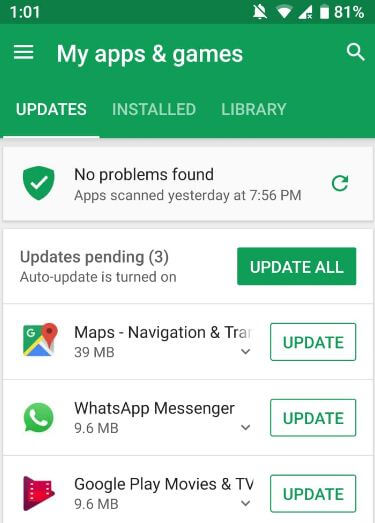This is a digital screenshot taken at 1:01, showing an 81% battery level. The main screen displays various apps and games, along with a search option. A navigation bar includes options for 'Updates', 'Installed', and 'Library'. A notification at the top states "No problems found, apps scanned yesterday at 7:56 PM," and features a green refresh button on the right and a green shield with a white checkmark symbol on the left. Below this, the message "Updates pending (3)" is displayed, with 'Auto-update' turned on.

A prominent "Update All" button, colored green and white, is visible. Individual app update options are shown below, including:
- Google Maps with a 'G' logo and a red pin, accompanied by an 'Update' button.
- WhatsApp Messenger, featuring a green and white logo with an old-fashioned telephone icon, also with an 'Update' button.
- Google Play Movies & TV, which also has an 'Update' button next to it.